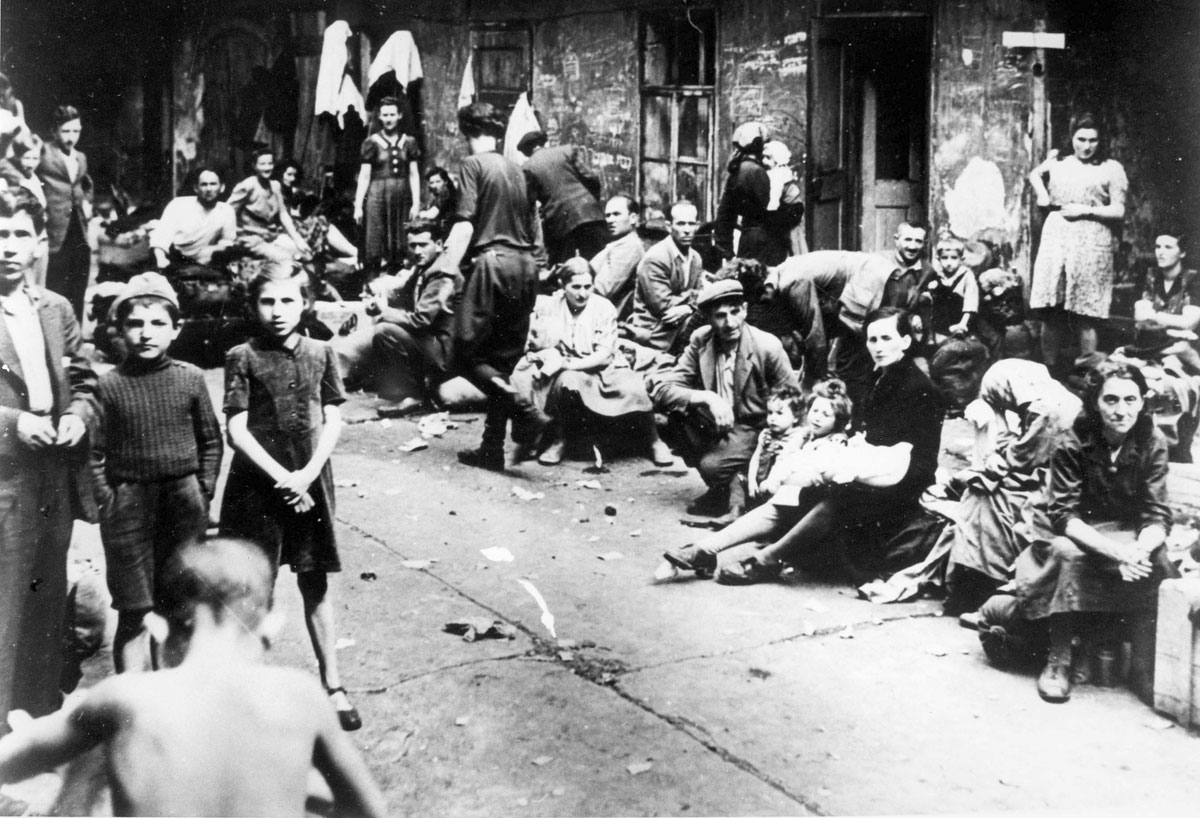In this striking black and white photograph, a large group of people is captured in anticipation, seemingly waiting outside. The mixed crowd includes children, men, and women, all clad in clothing characteristic of the 1930s or 1940s, suggesting a historical context. Many individuals are seated on the ground, while others stand, creating a dynamic composition of diverse postures. In the background, an old building with visible white markings and an open door on the right side looms above the crowd, adding to the scene's vintage atmosphere. The ground beneath them is worn concrete, indicative of its age, with varying degrees of wear and texture. In the bottom left-hand corner of the photo, a young boy, shirtless and bald, stands out. He faces away from the camera, revealing the top of his back and the crown of his head, adding a poignant human element to the scene.